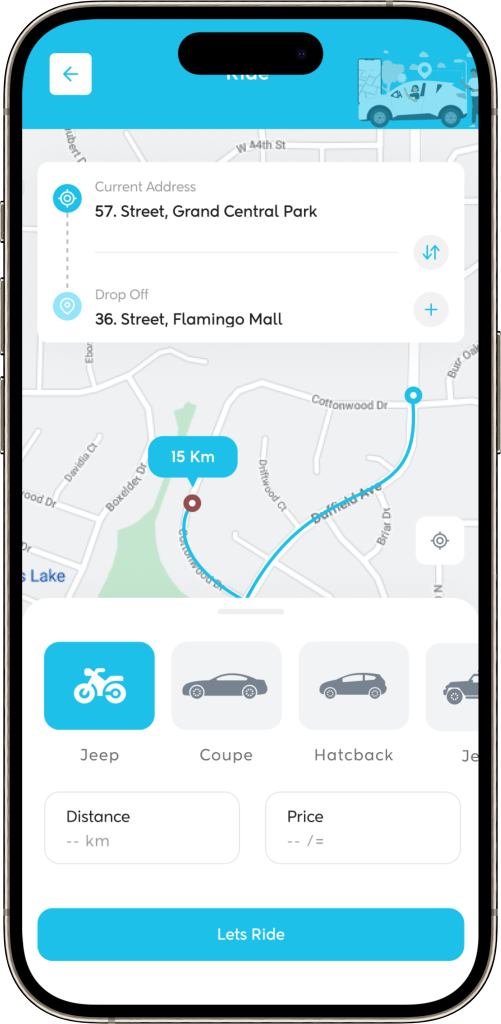The image depicts a mobile phone screen displaying a navigation app. On the right side of the phone, the power button is visible, while the volume up and volume down buttons are on the left. There is also a port or switch, possibly for a headphone jack or silent mode. At the top of the screen, the background is a bright light blue. In the upper-left corner, a white square with rounded edges contains a blue left-pointing arrow, partially obscured by the speaker area. Next to it, in the upper right section, there appears to be an icon or sign.

The screen transitions to a light gray map featuring a route highlighted in bright blue. A comment bubble with a blue background displays "15KM" in white text. Overlaying the map at the top is a white rectangular box; the top line in gray reads "current address," and below in larger black font, "57. Street, Grand Central Park." To the left of this address, there's a white compass icon set against a blue circular background. Gray dots descend from the compass icon, leading to a light blue circle with a white map pin in its center.

Adjacent to this, in small gray text, it says "drop off," followed by "36, Street, Flamingo Mall" in black font below. On the right side of the screen are two circular icons: The top one is a gray circle with blue arrows pointing up and down, and the bottom one is a gray circle featuring a blue plus sign in the center.